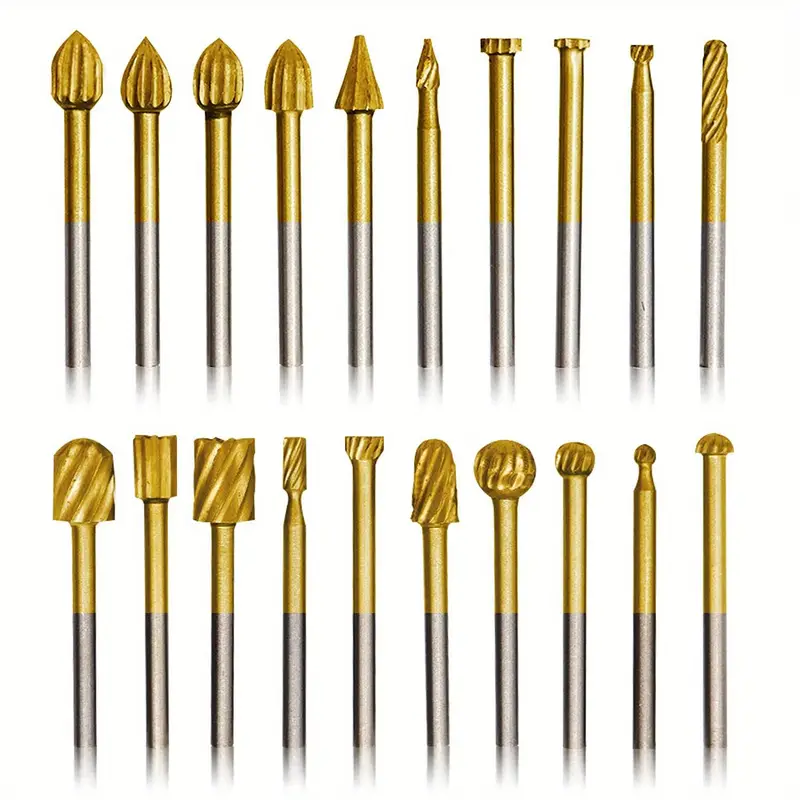The image depicts a collection of 20 intricately designed tools, possibly drill bits or specialized boring tools, arranged in two rows of ten each. Each tool features a two-toned shaft—silver at the bottom transitioning to gold at the top—culminating in a gold tip with varying shapes. These shapes include a range of spearheads, some flat and others notched, as well as rounded balls that taper from larger to smaller sizes, teardrop shapes, and even twisted patterns that could be used to create decorative grooves. The tools are vertical, appearing as if displayed in a tool set, and demonstrate a diverse array of tips likely intended for detailed work in materials such as wood or metal.